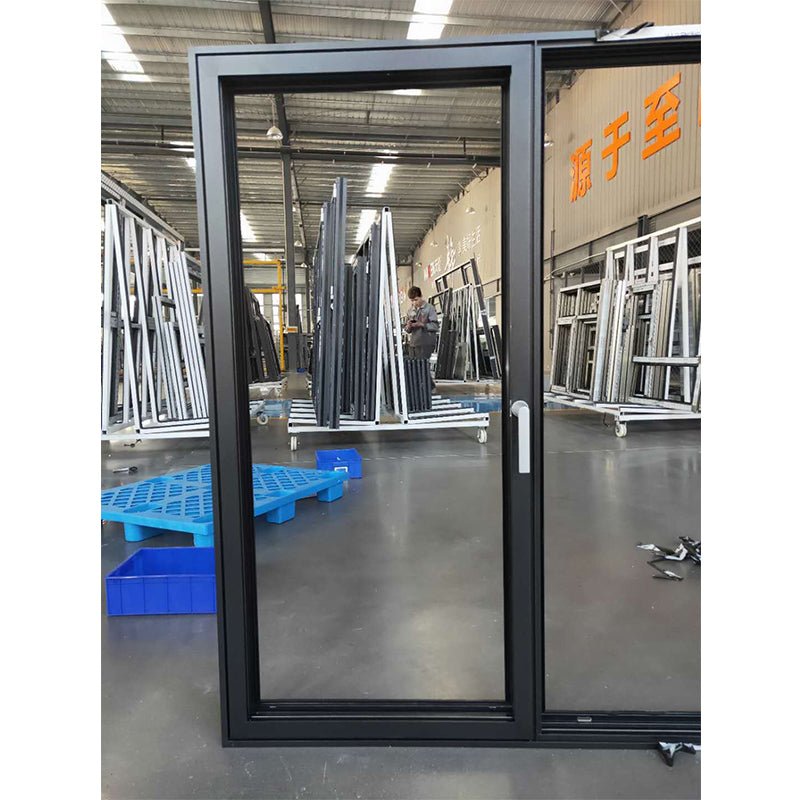The photograph captures an indoor factory scene that manufactures doors and windows. The image is rectangular with the longer sides on the left and right. The space is illuminated by large fluorescent lights mounted on the ceiling. In the background, rows and stacks of aluminum doors are positioned on their sides atop pallets and metal racks. Dominating the foreground is a black metal door featuring a white handle located on its right side. The door itself is rectangular, with a rectangular opening for an additional glass panel also on the right. Behind this door is a tall metal wall adorned with orange Chinese characters, indicating that the factory may be situated in an Asian country.